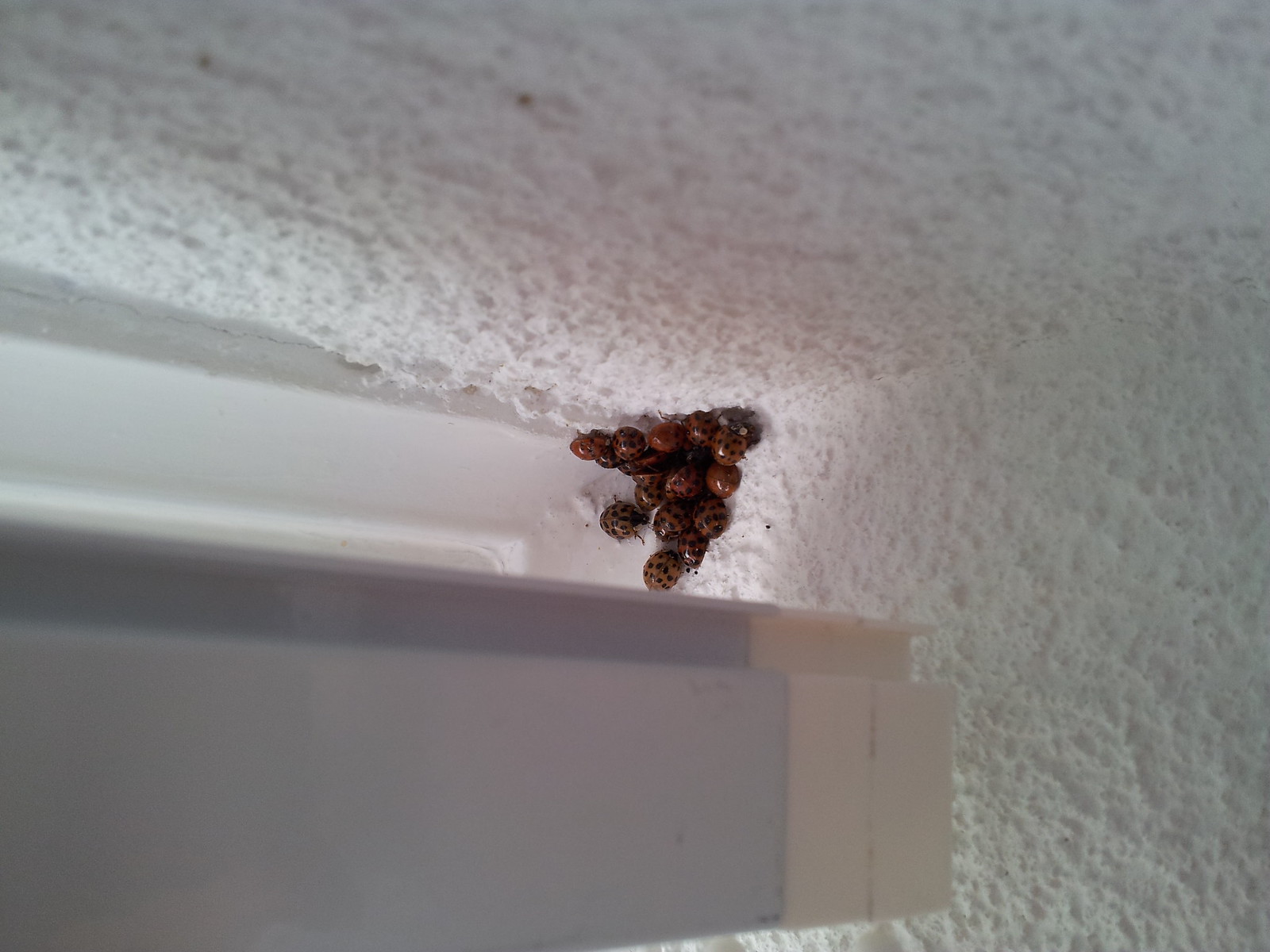The photograph captures a close-up view of a textured white wall and ceiling corner, resembling a popcorn finish. In the image's center, a cluster of approximately 20 ladybugs of varying shades of red, some even orange or yellowish, are tightly gathered. These ladybugs, each adorned with black spots that differ in number, are stacked upon each other in the corner where the wall meets the ceiling. A light silver metal rail, potentially part of a window frame or curtain rod, extends into view, adding to the context of an interior setting. The overall scene is intriguingly detailed, with the soft whites of the walls contrasting against the spotted red bodies of the ladybugs.